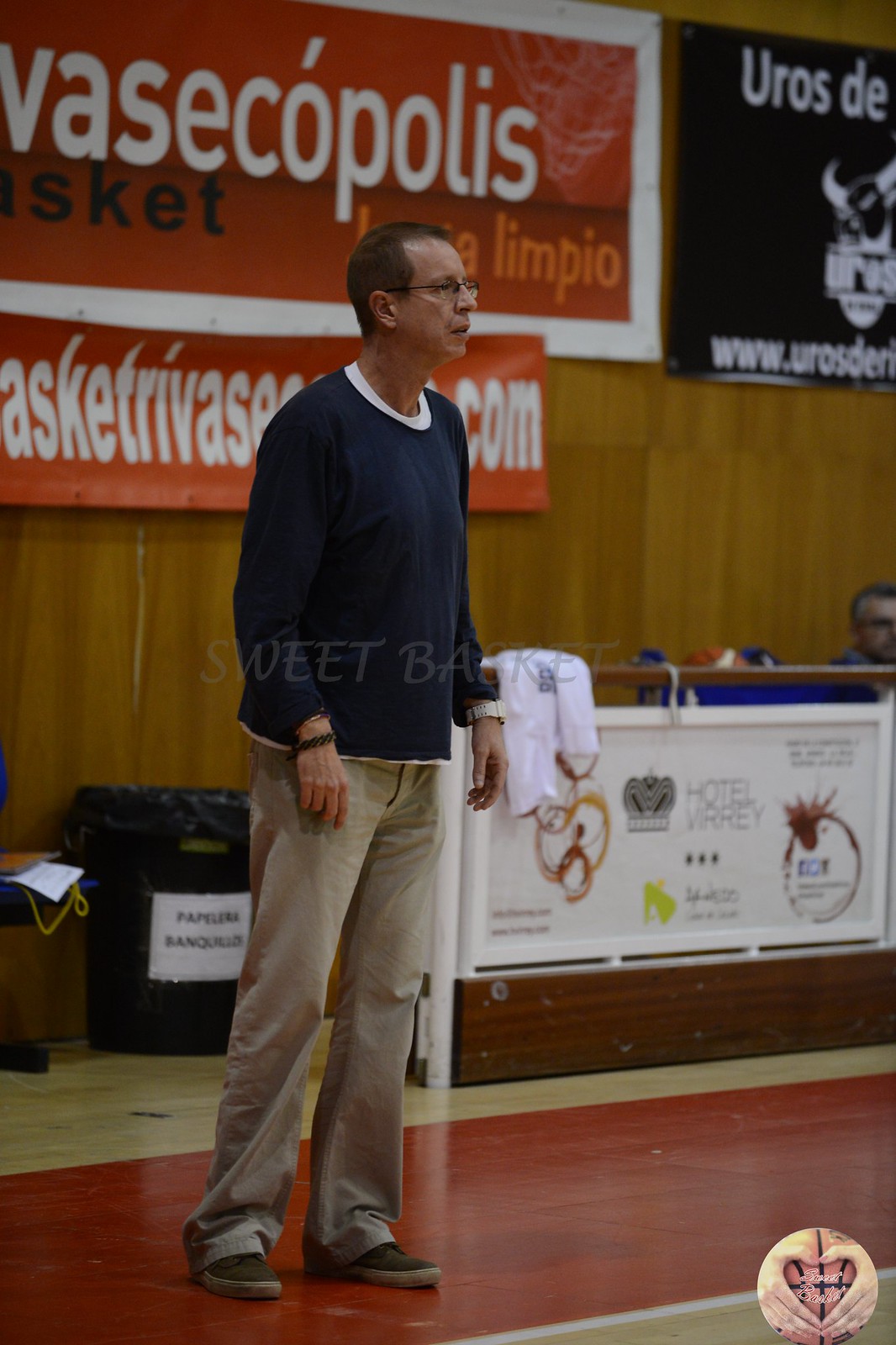In this detailed photograph, a man is positioned slightly left of center, looking intensely to the right, possibly towards referees. He is dressed in a stylish blue sweater layered over a white shirt, paired with tan khaki pants and fresh brown shoes. He accessorizes with a wristband on one hand and a white-strapped watch on the other. The man, who has very short hair and glasses, stands on a gymnasium floor featuring a light wood finish with a red stripe outlined in white. 

Behind him, the left side of the image shows a brown wall adorned with several large banners. These banners predominantly showcase reddish-orange colors with white, orange, and black text, while the topmost one has a white outline. There is also a black banner with white writing and a symbol, although it becomes blurry at the edge of the frame. At floor level, a small black trashcan with a white sign is visible. On the right side of the image, there's a long podium adorned with various announcements and symbols. Extending off the right edge of the podium, half of a man's face is partially visible from the chin up. The gymnasium's white and red court extends into the very bottom right corner, where a round symbol can also be seen.